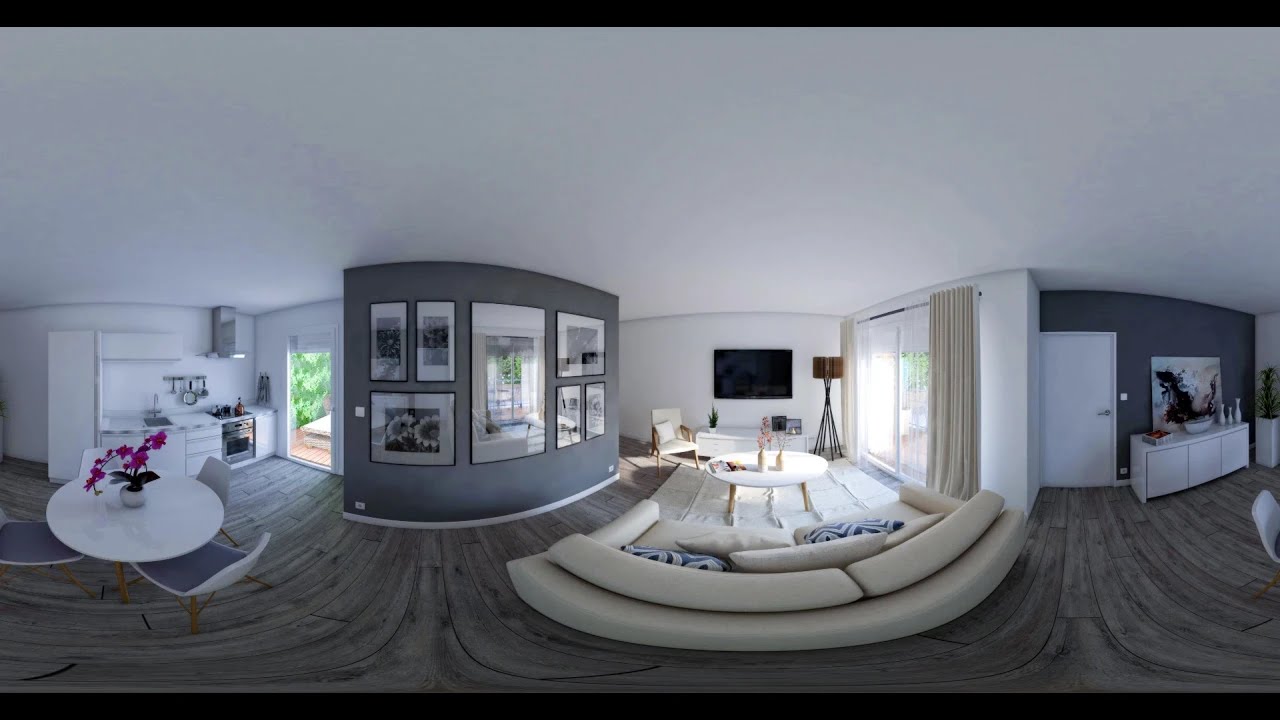The image presents a panoramic and somewhat distorted view of the interior of a modern home. At the center, the living room features a beige couch facing a circular white coffee table set on a white rug. Positioned in front of the coffee table is another square table, and to the left of this setup, there is a white armchair adorned with a small white pillow. Just beyond the seating area is a TV mounted on the back wall, accompanied by a white console table underneath it and a tall, intricate lamp situated to the right of the TV.

To the right side of the photo, there are large sliding glass doors emitting natural sunlight, framed by subtly tan curtains. Adjacent to these doors is a sophisticated white entry door flanked by a modern white entry console table.

On the far left side of the image is an open kitchen area, characterized by its sleek, white design. This space includes a white dining table with three chairs encircling it, and a vibrant pink flower arrangement in a white pot at its center. The kitchen's background reveals an array of appliances, countertops, and hanging utensils, with a gray accent wall displaying panoramic photos.

The flooring throughout the image is a gray plank, and the ceiling is painted white, complementing the predominantly white and gray color scheme of the interior.